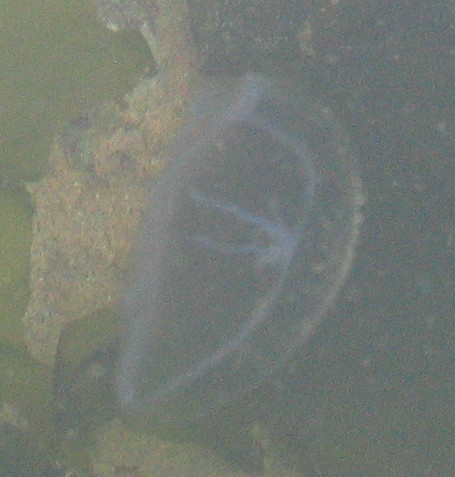The image appears to capture an underwater scene characterized by a murky, greenish hue that permeates the entire photograph. Predominantly to the left, the terrain takes on a flat, sandy appearance. Central to the image is a somewhat oval-shaped, translucent object with blue-tinted, finger-like projections radiating from its middle. Though the object resembles a jellyfish or a see-through plant, the image’s blurriness leaves room for speculation. This oval entity sits against a textured, rocky surface. To the right, the scene fades into darker, murky waters, enhancing the overall mysterious and obscure quality of the photograph.